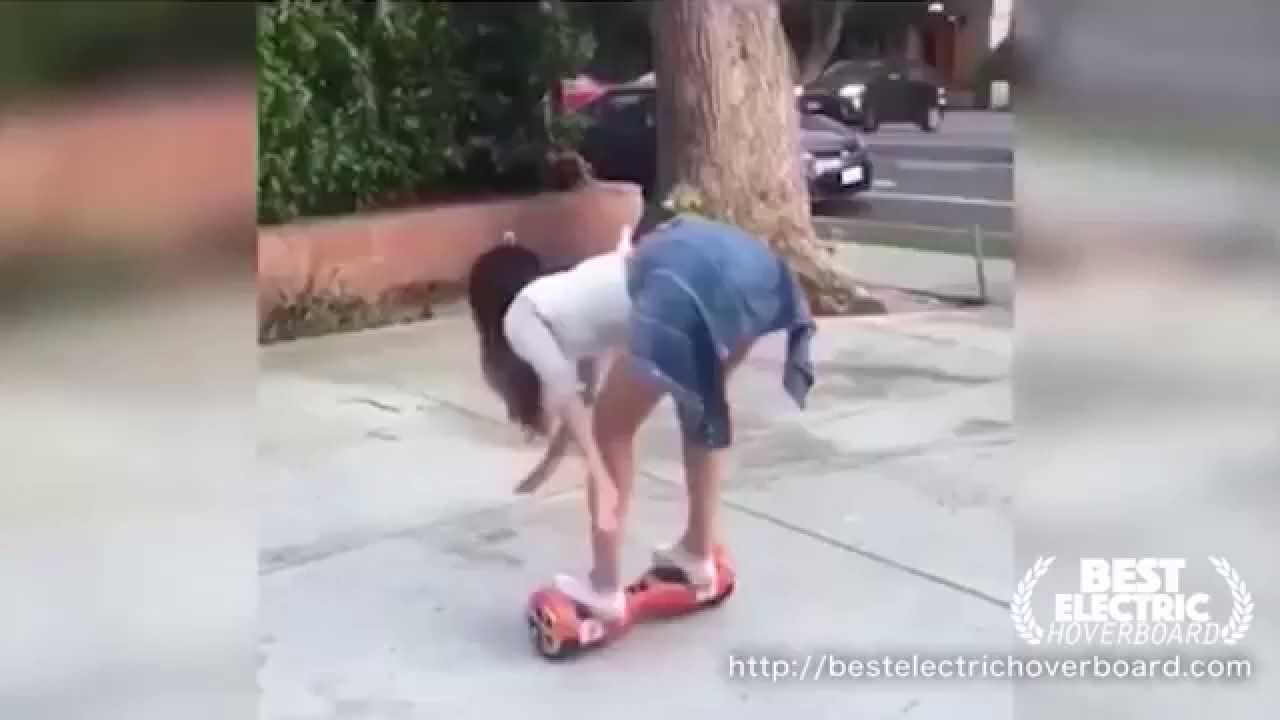A young girl with long, dark hair is riding a red hoverboard on a concrete driveway. She is wearing a white long-sleeved shirt with the sleeves casually pushed up to her elbows, and a blue jacket tied around her waist. Her legs are bare except for a pair of socks. She is captured bending forward slightly while balancing on the hoverboard. In the background, there is a car driving by on the street, with a truck visible further in the distance. The top left corner of the image features a thick, impenetrable hedge sitting atop a concrete wall. An inscription at the bottom right corner reads "Best Electric Hoverboard," followed by a URL: "http://BestElectricHoverboard.com."